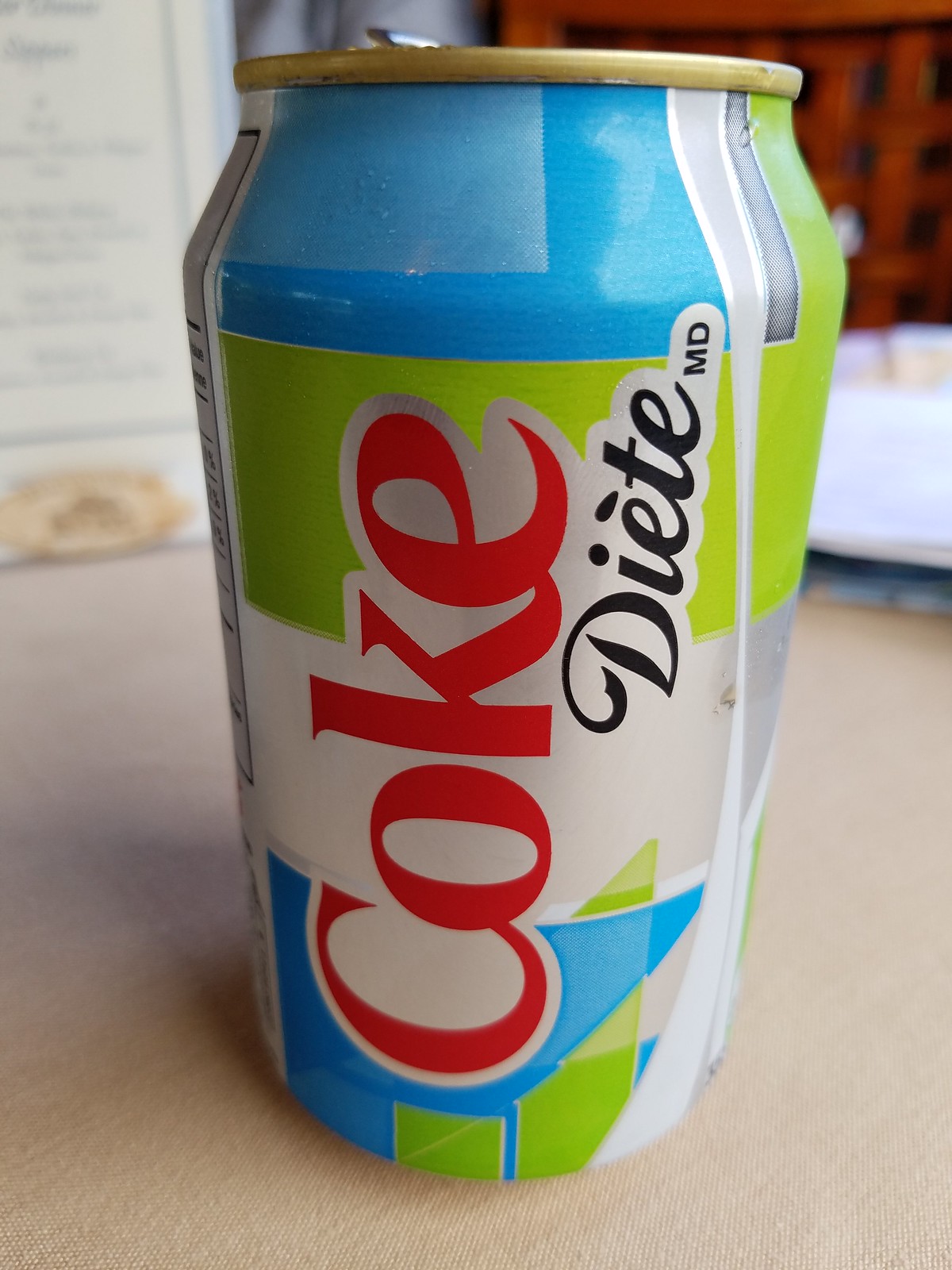The image features a uniquely designed Coke can captured from a side angle, showcasing its full side profile while leaving the top out of view. The can rests on a plush brown carpet, which adds texture to the foreground. In the background, a blurred bed and wall can be discerned, providing context to the indoor setting. Unlike the classic Coke can, this one features a striking design with a blue top. A green stripe encircles the can, ascending towards the top. Below the green stripe, a section of unpainted silver metal is visible, further complemented by more blue at the bottom and additional green accents. A vertical silver stripe runs along the entire height of the can. Bold red letters spell out "C-O-K-E" vertically from bottom to top, drawing immediate attention. To the right of this, the word "diet" is written in elegant black cursive, followed by the initials "M-D" in the same style, adding a personalized or possibly regional touch to the can's design.